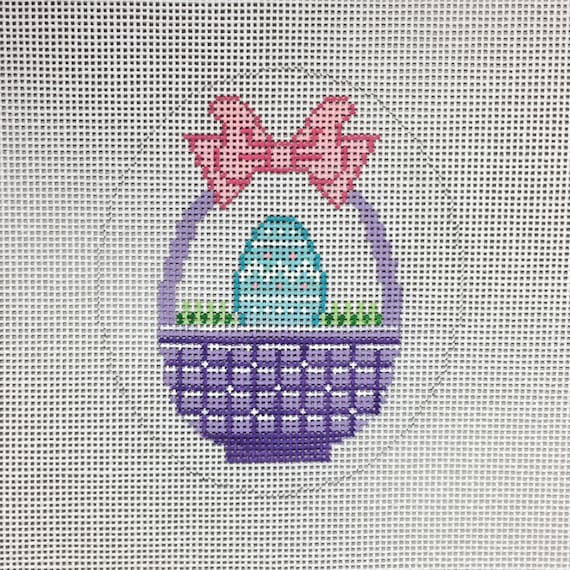This image showcases a detailed cross-stitch pattern featuring a traditional Easter theme. At the center of the design is a lavender woven Easter basket adorned with a pink bow on its handle, complete with darker purple cross hatching to mimic the texture of a real basket. Inside the basket sits a turquoise Easter egg with pink polka dots and white zigzag patterns, nestled in a bed of green Easter grass depicted with dark and light green threads. The entire scene is framed within an egg-shaped light gray oval that contrasts against a dotted purple background. The meticulous craftsmanship suggests that significant time and care have been invested, evoking a charming, country-style aesthetic reminiscent of handmade heirlooms.